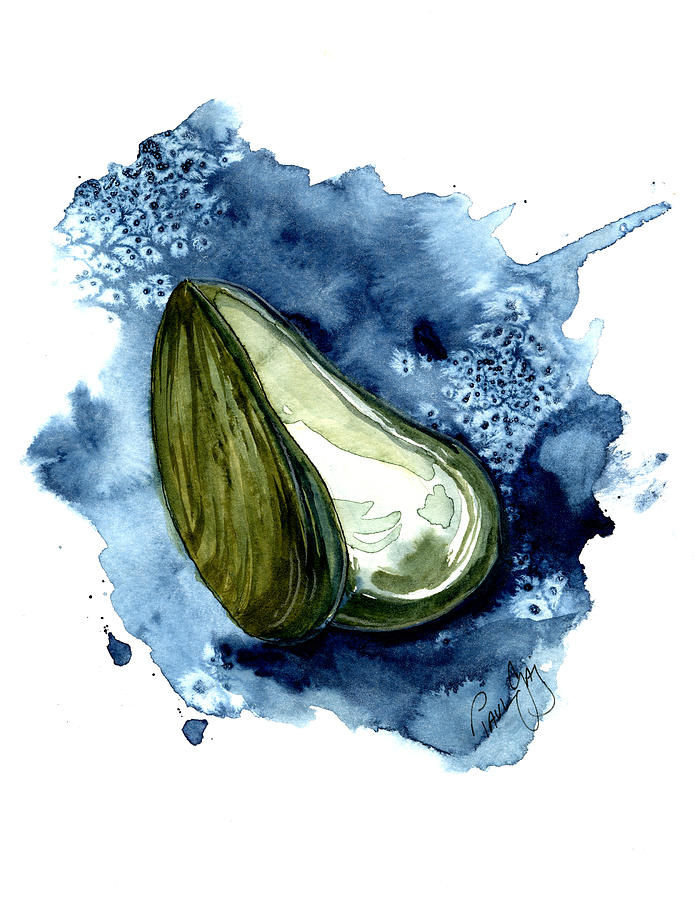This is a detailed watercolor painting of a clam with an open shell. The exterior of the shell displays swirling stripes of green, gray, and black, while the interior reveals a milky white surface with a greenish hue starting from one side. The clam is set on an abstract puddle of water in varying shades of blue and white, which features tiny, delicate white flowers resembling dandelions with black centers. The background is a mix of blues, including dark blue, light blue, navy, and baby blue. The painting is signed at the bottom in black lettering by Laval J. Additionally, there are small, barnacle-like shapes scattered on the blue surface.